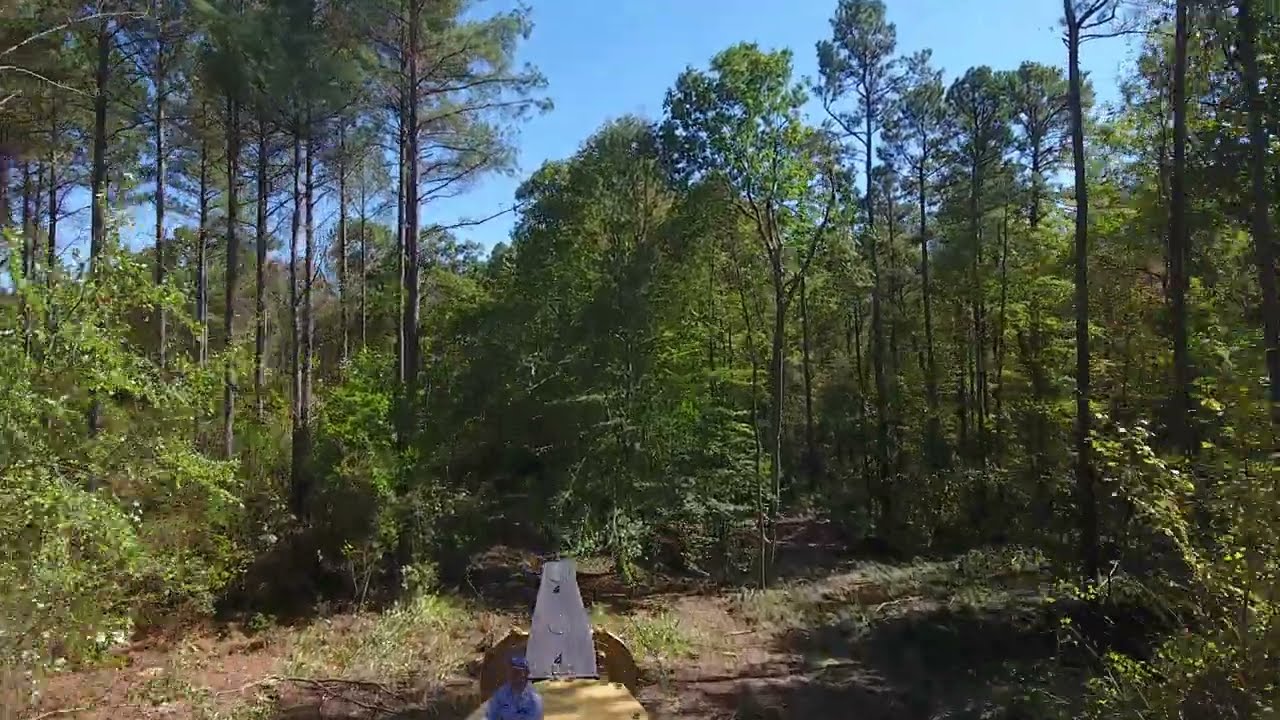In this horizontally aligned, rectangular image set in a desolate, heavily treed forest area, the top quarter reveals a clear blue sky without any clouds. Tall, narrow tree trunks dominate the background, each crowned with green leaves. The lower half of the image shows a ground covered in brown dirt, tall grass, various types of plants, and scattered tree branches. At the very bottom, slightly blurry but prominent, stands a person whose gender is indeterminate. They are wearing a long-sleeved blue shirt and a blue hat, appearing to be on or near a yellow platform or wooden plank with a vertical white piece attached to the back. Despite the person being the closest element to the camera, the overall poor image quality makes further details difficult to discern, but the scene is clearly bathed in daylight. No text is visible anywhere in the picture.